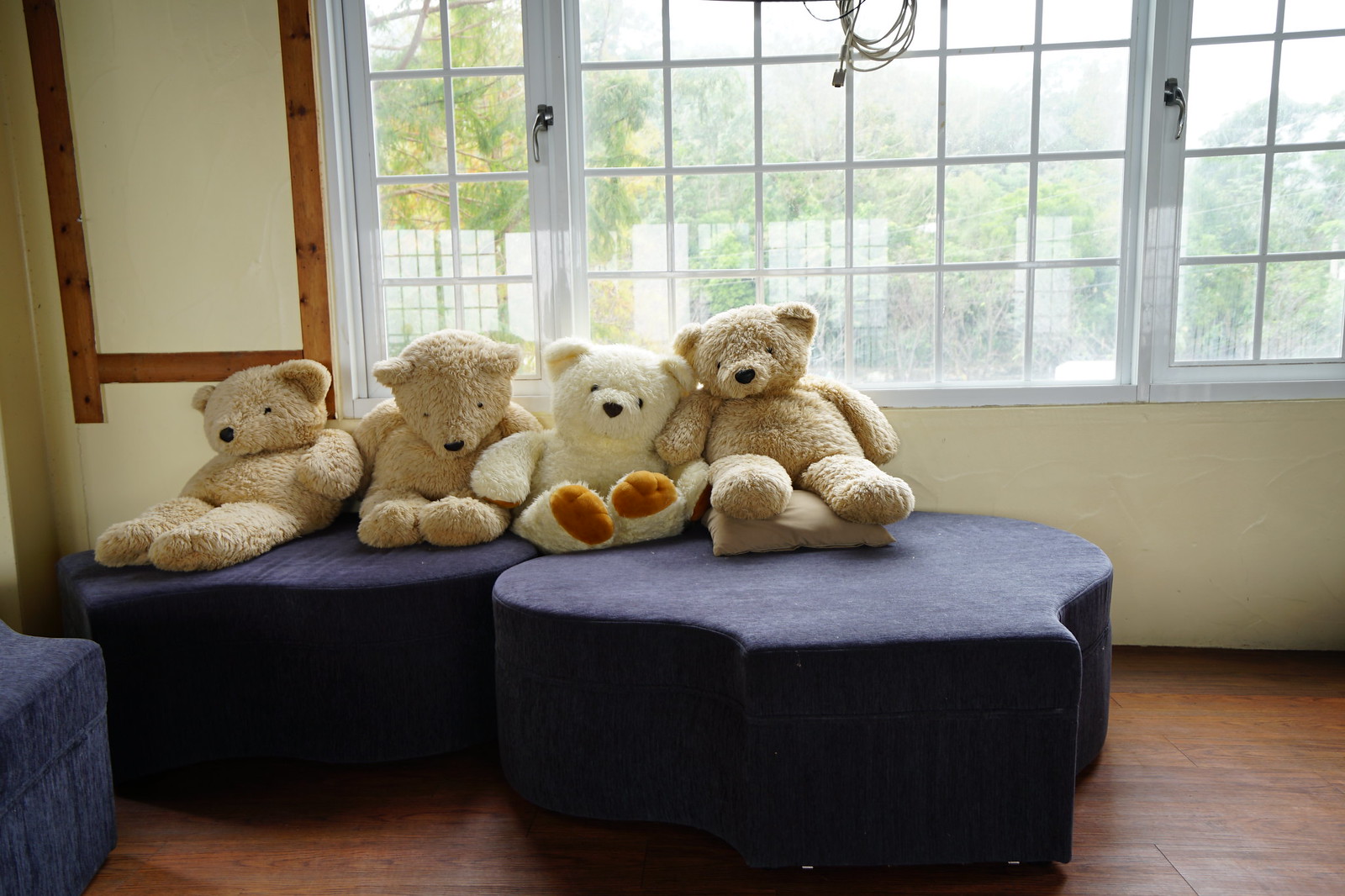The image captures an inviting indoor scene with four fluffy teddy bears arranged on sturdy, deep blue ottomans that resemble large denim-inspired seating. These ottomans, with their firm and flat surfaces, support the teddy bears, which have big ears and varying facial expressions. Three of the bears are a light brown, while one stands out as white with brown paws, adding a touch of variety.

Behind the bears, a large bay window composed of multiple smaller square panes and framed in white dominates the background, allowing ample light to flood the space. The bay window, with its white border, offers a picturesque view of trees and greenery outside. Additionally, there are two side windows, one on the left and one on the right, each equipped with handles to open inward, contrasting with the fixed central bay window. The windows are set into white walls adorned with wooden frames, subtly enhancing the cozy interior. A piece of furniture, possibly a sofa matching the blue ottomans, peeks in from the bottom left corner.

A cable hangs from the ceiling in the upper right of the photo, adding a slight, intriguing disruption to the overall serene and organized setting. An elegant whiteboard encased in a brown frame is mounted on one wall, blending seamlessly with the room's warm and inviting aesthetic. The dark wooden floors further complement the tranquil atmosphere of this charming space.